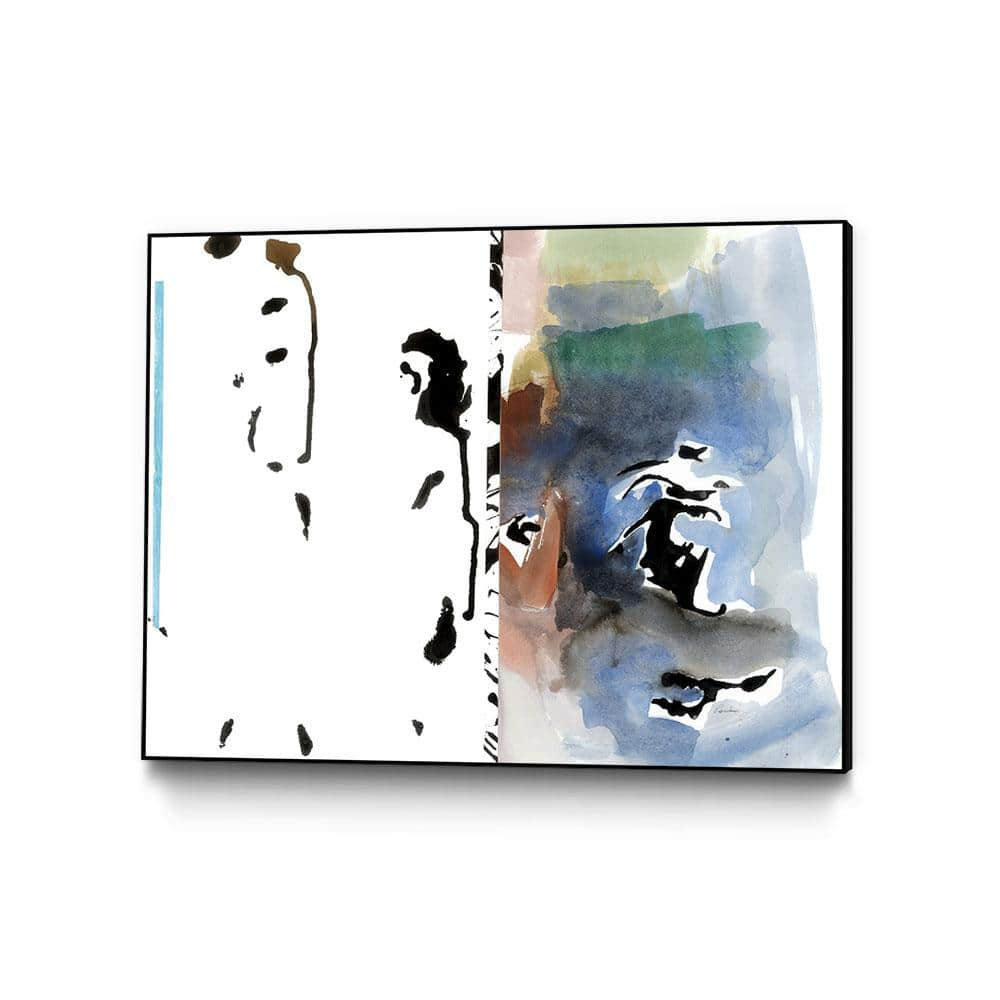This piece of abstract impressionistic art features a rectangular shape with a subtle black frame that gives it a slight three-dimensional effect as it hangs on a white wall, casting delicate shadows. The composition is distinctly divided vertically into two contrasting sections. The left-hand side predominantly showcases a minimalistic white background adorned with an array of black and light brown ink blobs or splotches, resembling fingerprints or silhouettes. Among these shapes, a vertical light blue line runs parallel to the left border. In stark contrast, the right-hand side bursts with more vibrant yet muted watercolor hues—comprising blues, greens, pinks, and browns—partially obscuring the white background. Central to this side, amidst the colorful backdrop, are abstract black shapes, potentially mimicking the form of a person standing on a rock. This complex interplay of colors and forms creates a visually striking juxtaposition between simplicity and intricacy.